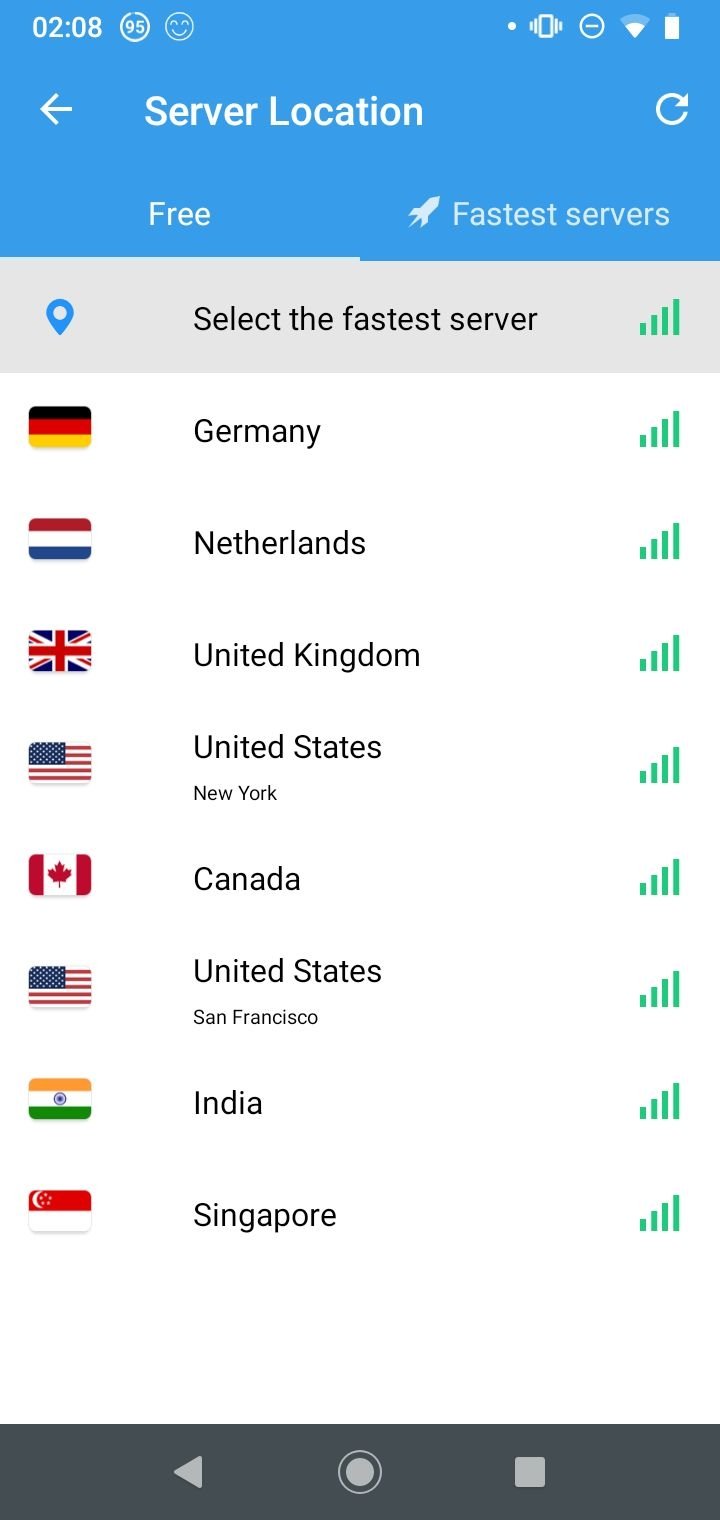This screenshot, taken on a smartphone, features a user interface with various details visible. In the top-left corner, the timestamp "2:08" is displayed alongside two logos which are unrecognized. All this information appears in white text. The top-right corner shows the battery percentage, Wi-Fi signal strength, and a few other icons, all set against a blue background occupying roughly the top 15% of the screen.

On the left side of this blue section, the text “Server Location” is prominently displayed in white. To the left of this text is a left-pointing arrow. Below it, the word "Free" is visible, followed by a small white rocket icon in the bottom right corner of the box, with "Fastest Servers" stated next to it.

The main portion of the screenshot, below this blue header area, lists eight available Wi-Fi server options, each named after a different country: Germany, the Netherlands, United Kingdom, United States, Canada, United States (listed again), India, and Singapore.